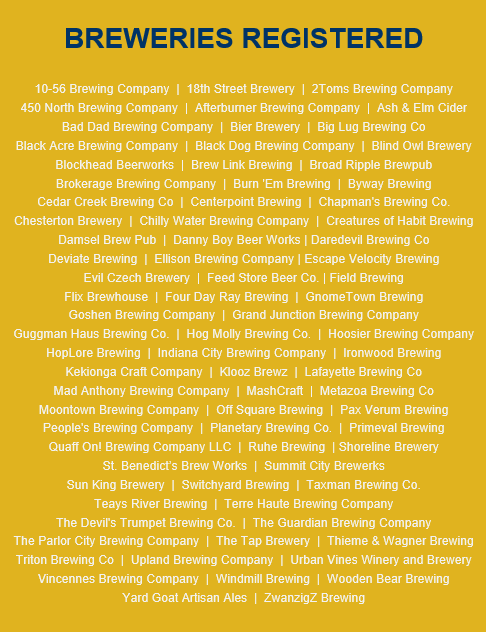The image features a printed sign with a gold background and dark blue and white text. At the top, in dark blue, block capital letters, the title reads "Breweries Registered." Below this title, an extensive alphabetical list of brewery names begins with numerals and continues through the alphabet, ending with the letter Z. Each name is printed in white. The names range from "1056 Brewing Company," "18th Street Brewery," and "2 Toms Brewing Company" to "Zwanzig Brewing." The list is detailed, with most lines containing three brewery names unless space constraints due to longer names limit it to two names per line. Although the list primarily uses white text, the gold background enhances legibility and adds a touch of elegance to the sign. Overall, the sign meticulously catalogs numerous breweries in a structured and visually appealing manner.